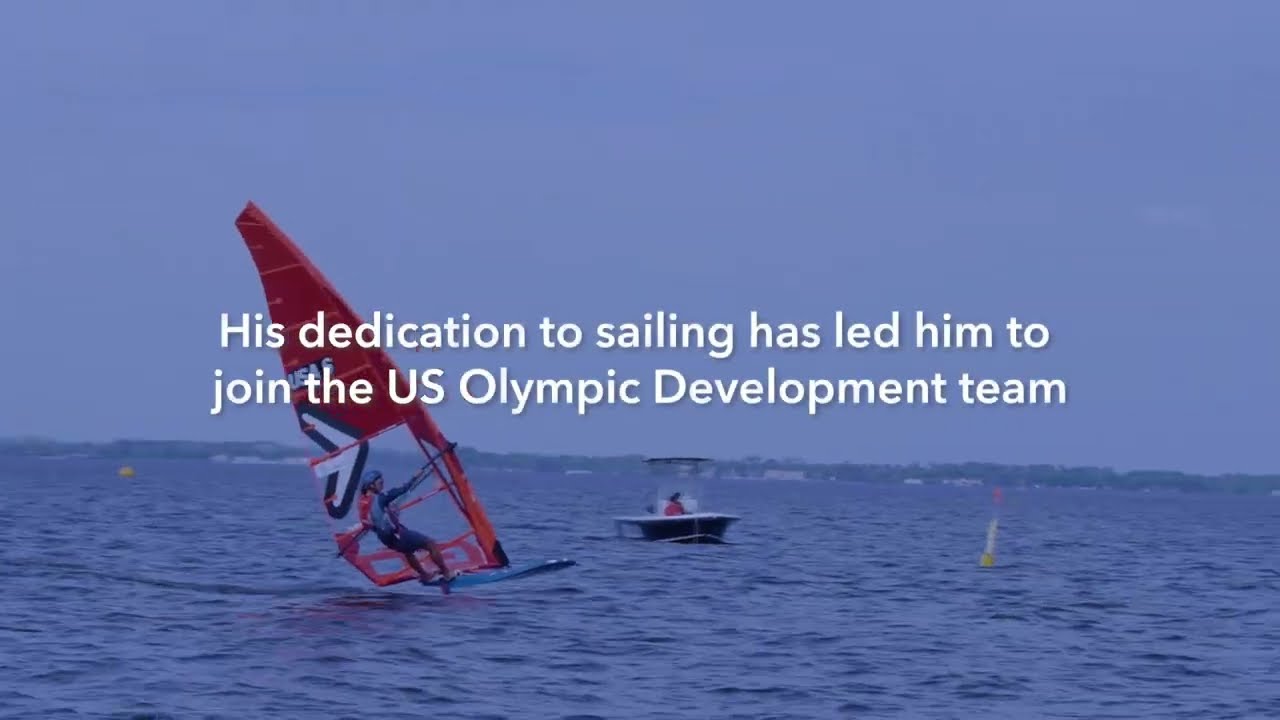In the photograph, an Olympic-level windsurfer is captured navigating the ocean waters under a cloudy yet bright sky. The windsailer, adorned in a black wetsuit with blue accents and a matching blue helmet, is skillfully leaning back on his purple windsurfing board with a red sail. The image prominently features white text in the center, proclaiming, "His dedication to sailing has led him to join the U.S. Olympic development team." Positioned slightly to the left within the frame, the windsurfer is the focal point, clearly demonstrating his prowess and commitment. A low-level motorboat, likely supervising his training, is visible in the background along with a distant strip of land and a yellow buoy. The dark blue ocean waters have gentle waves, adding a dynamic element to the scene. This inspirational image, potentially part of a promotional campaign, aims to motivate viewers to consider sailing and recognize the dedication required to reach the Olympic level.